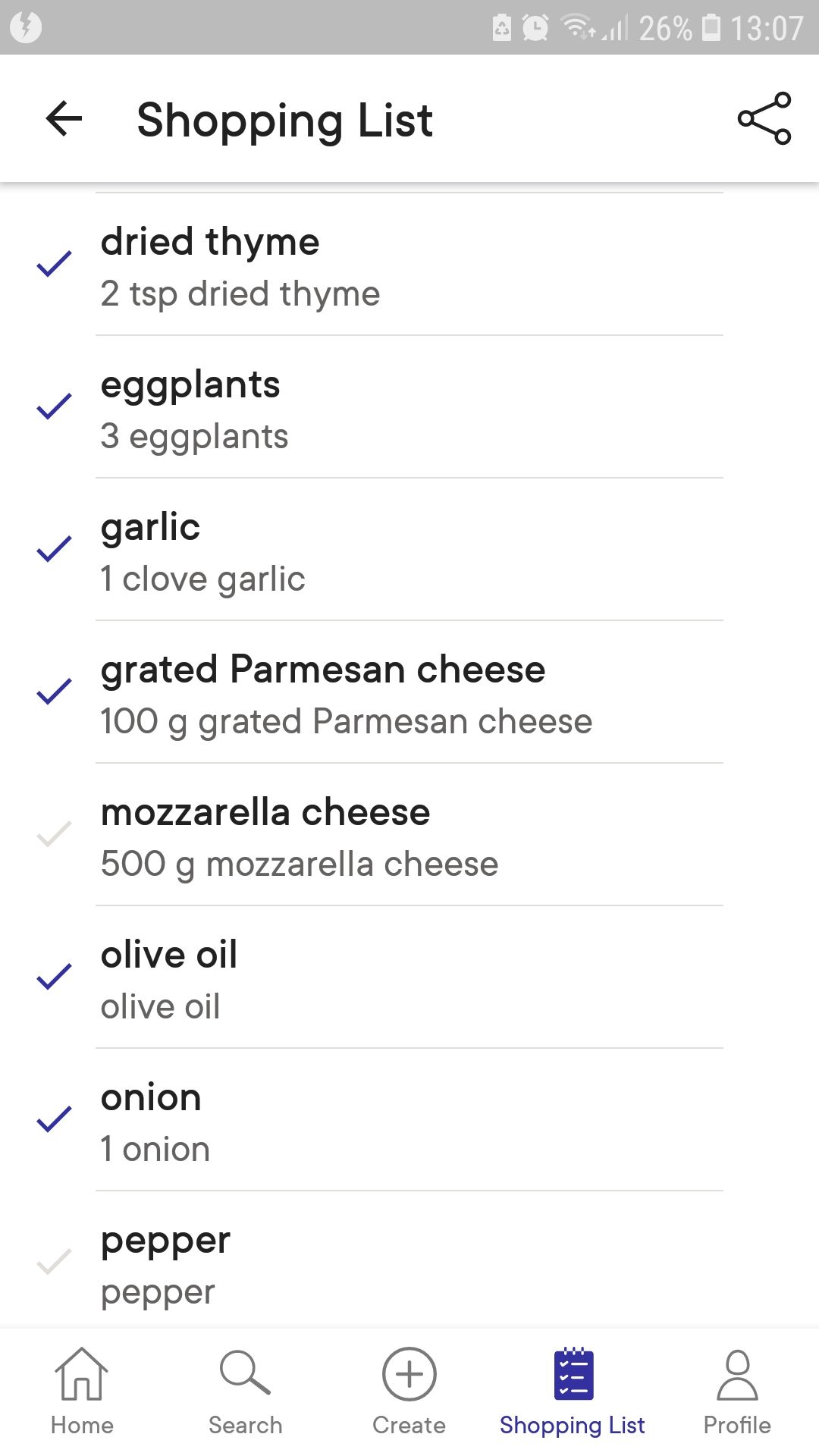This screenshot captures the display of a mobile device, specifically showcasing someone's digital shopping list. The interface is simplistic, featuring a stark white background and devoid of any colorful elements, images, or decorative icons. At the very top, a gray taskbar houses standard mobile device icons, including indicators for battery life, time, cellular signal strength, and Wi-Fi connectivity.

Dominating the screen is the user's shopping list, identified clearly at the top of the page. This functional layout lists several grocery items, each accompanied by a checkbox indicating their acquisition status. The items and their details are as follows:

- **Dried thyme:** 2 teaspoons (Checked)
- **Eggplants:** 3 units (Checked)
- **Garlic:** 1 clove (Checked)
- **Grated Parmesan cheese:** 100 grams (Checked)
- **Mozzarella cheese:** 500 grams (Unchecked)
- **Olive oil:** No specified amount (Checked)
- **Onion:** 1 unit (Checked)
- **Pepper:** No specified amount (Unchecked)

Each item on the list is methodically organized, providing a clear and efficient overview of the user's shopping needs and what has already been procured.